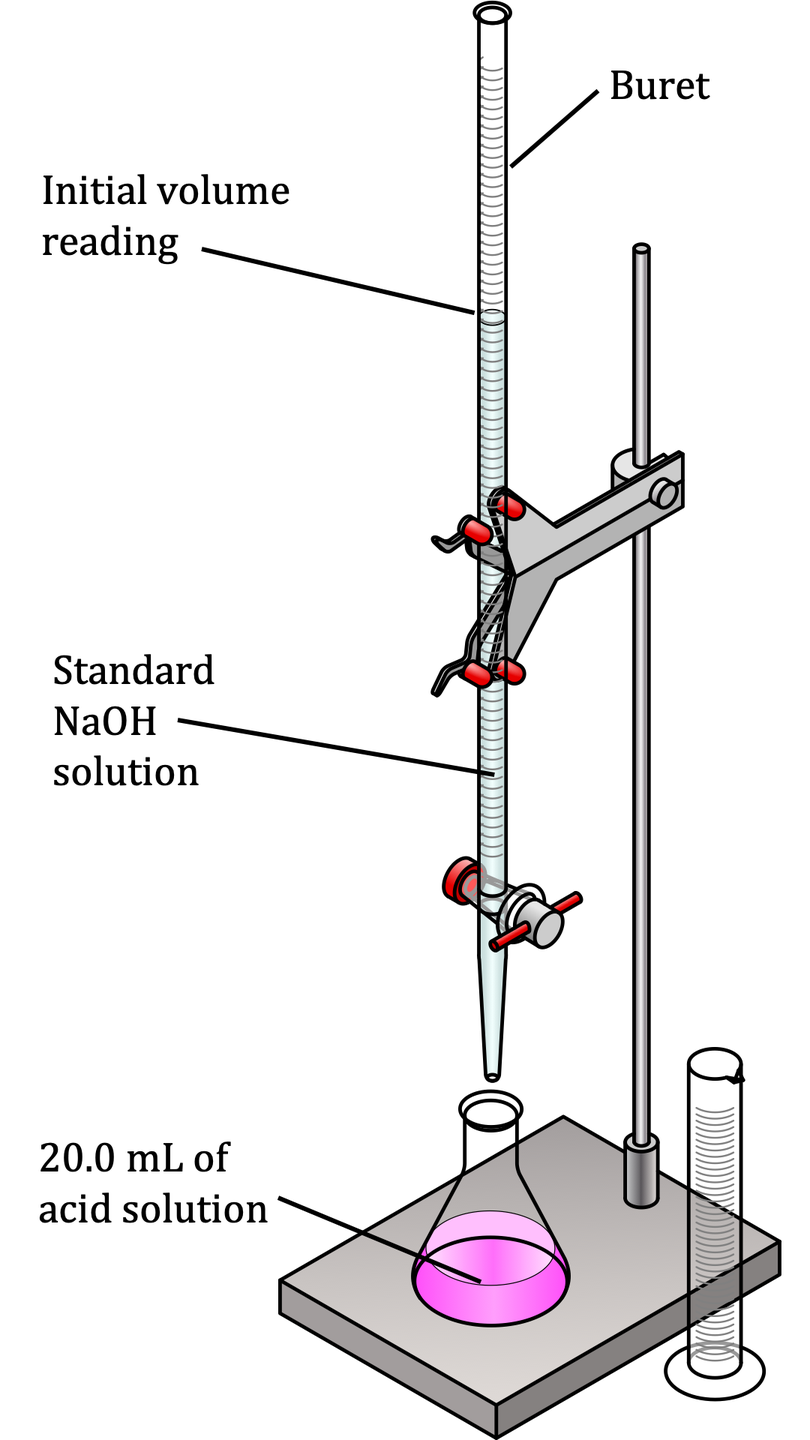The image depicts a detailed diagram of a chemistry experiment setup used for titration. In the center, there is a cylindrical beaker on a silver platform, containing a pink liquid labeled as "20.0 milliliters of acid solution." A long burette, held by a vertical stand with red clips, is positioned above the cylindrical beaker. The burette contains a blue liquid and has labeled markings for "initial volume reading" and "standard NaOH solution." Arrows and labels provide clear instructions on the procedure, indicating how the NaOH solution from the burette is to be gradually added to the acid solution in the beaker. Additional labels such as "Bure," and possibly "Bray" or "Britt," are noted, suggesting steps in the titration process to observe changes from the initial to the final volume readings.